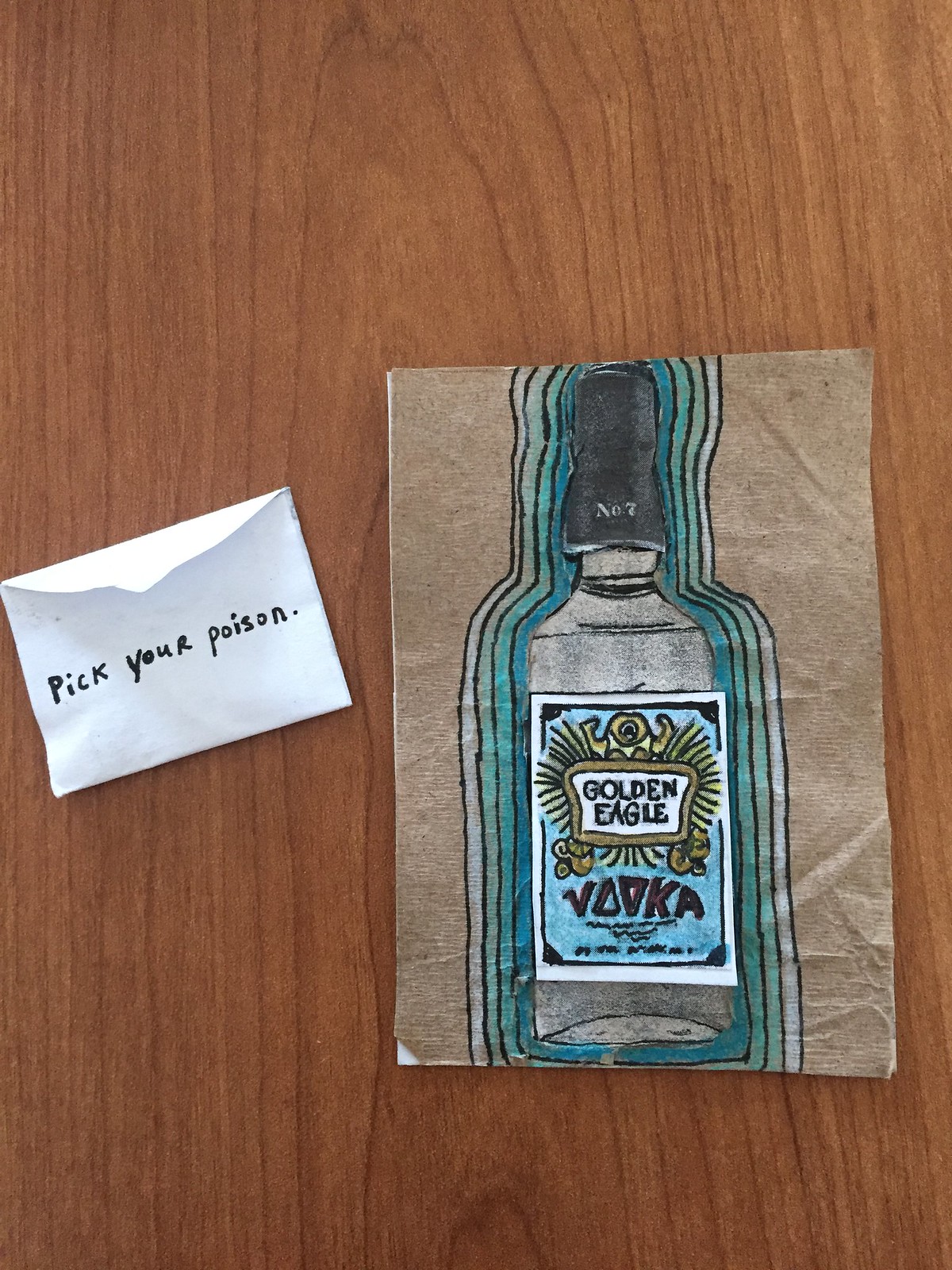In this detailed photograph set on a vertically-grained brown wooden table, we see an open white envelope on the left side with the hand-printed black letters reading "Pick Your Poison." The flap of the envelope is slightly ajar. Towards the right, there's a piece of thin, translucent paper displaying a detailed drawing of a vodka bottle. The label on the bottle reads "Golden Eagle Vodka" with a gold-bordered box and artistic strips hanging out from the sides. The bottle features a black handle and cap with a black number seven on it. The label is primarily blue with golden eagles on a white background, surrounded by expanding borders that transition through turquoise, aqua, gray, and white, giving a layered effect around the bottle illustration.